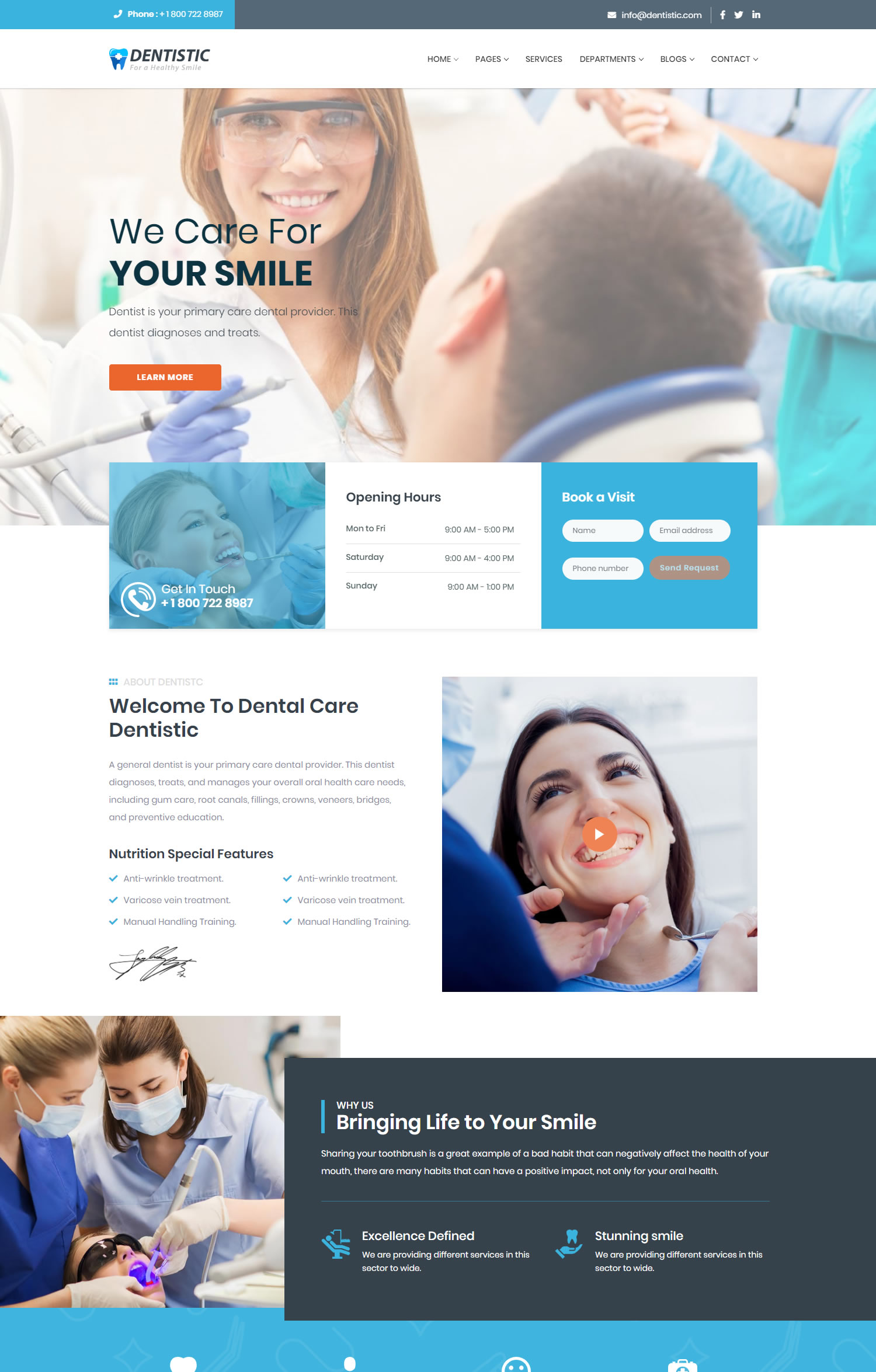The screenshot appears to depict the home page of a website likely named "Dentistic." At the top left, the word "Dentistic" is displayed in black capital letters, accompanied by a small, blue tooth icon. The upper left border of the page is blue, transitioning to gray for the remaining three-quarters. The background of the menu section is white, but the font is too small to read clearly.

Dominating the top of the page is a large photograph. It features a dental hygienist, a young white woman in her early to mid-twenties with reddish-brown hair, wearing safety glasses and a big smile. She has a blue glove on her right hand and is holding a dental instrument. Only the back of the patient's head is visible, revealing short brown hair.

Below this, there is a large square insert displaying what appear to be the clinic's opening hours, though the details are unreadable. The insert welcomes visitors with the text "Welcome to Dental Care Dentistic," followed by more text that is too small to decipher. To the right of this section, a video is indicated by a central play button icon. In the video preview, a smiling white woman with brown hair looks up at a hygienist, who is depicted partially, mainly showing a royal blue sleeve and shoulder.

At the very bottom of the page, a gray rectangle carries the slogan "Bringing Life to Your Smile" in white letters. To the left of this slogan is another photograph showing two white female dental professionals—one with blonde hair and the other with brown hair, both wearing surgical masks—working on a patient.